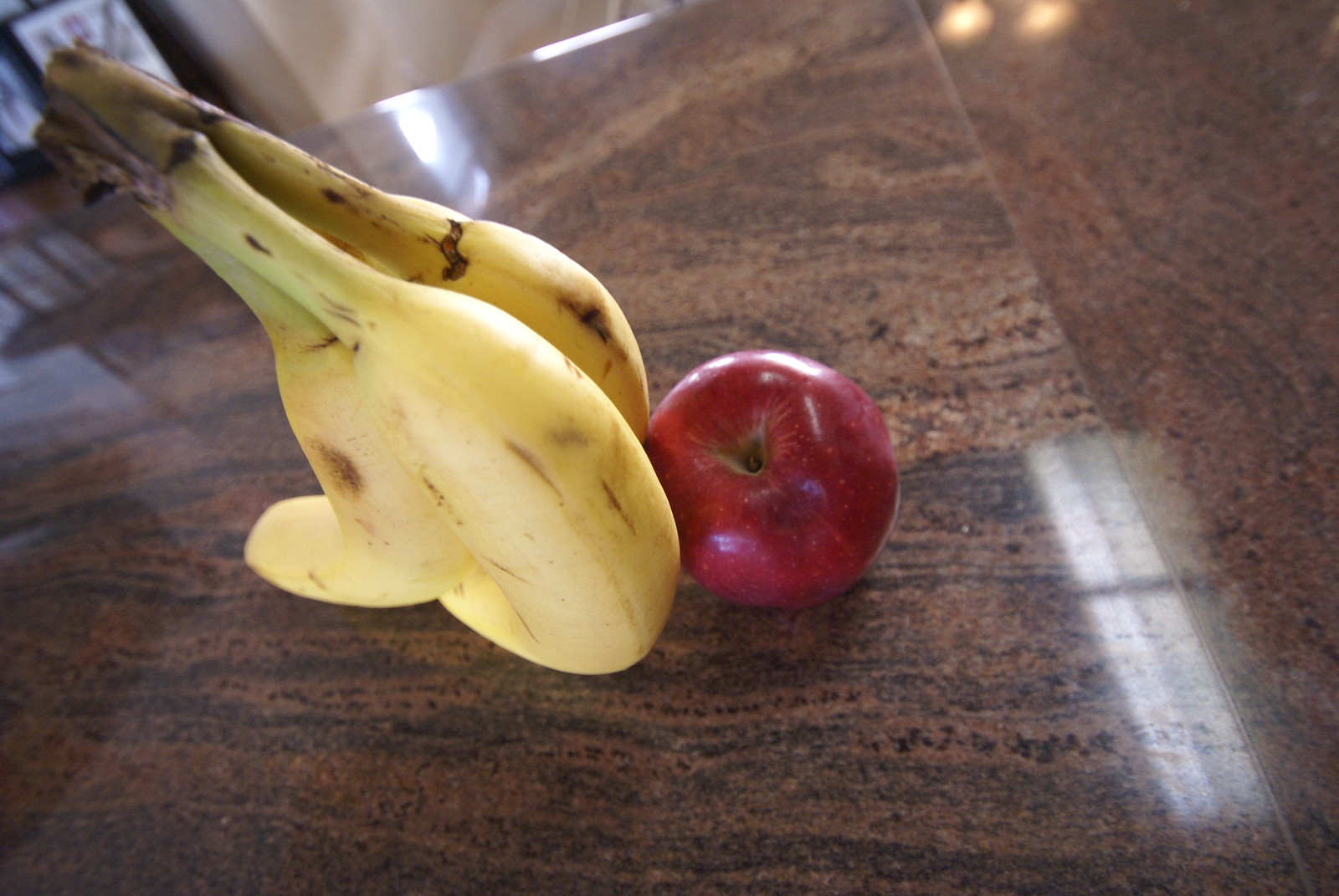Photograph of a highly polished kitchen work surface featuring a unique abstract wood effect in shades of brown and beige, with swirling patterns. The image employs a shallow depth of field, creating a blurred background that focuses attention on the objects in the foreground. In the top left corner, there's an indistinct image contributing to the overall aesthetic. Centered on the shiny surface are three bananas and a red apple. The apple, marked with a notable deep bruise, serves as the base against which two of the bananas are propped. Arranged in a somewhat artistic manner, the two bananas rest against the apple, while the third banana is positioned in front, acting as a stabilizer for this makeshift fruit sculpture.